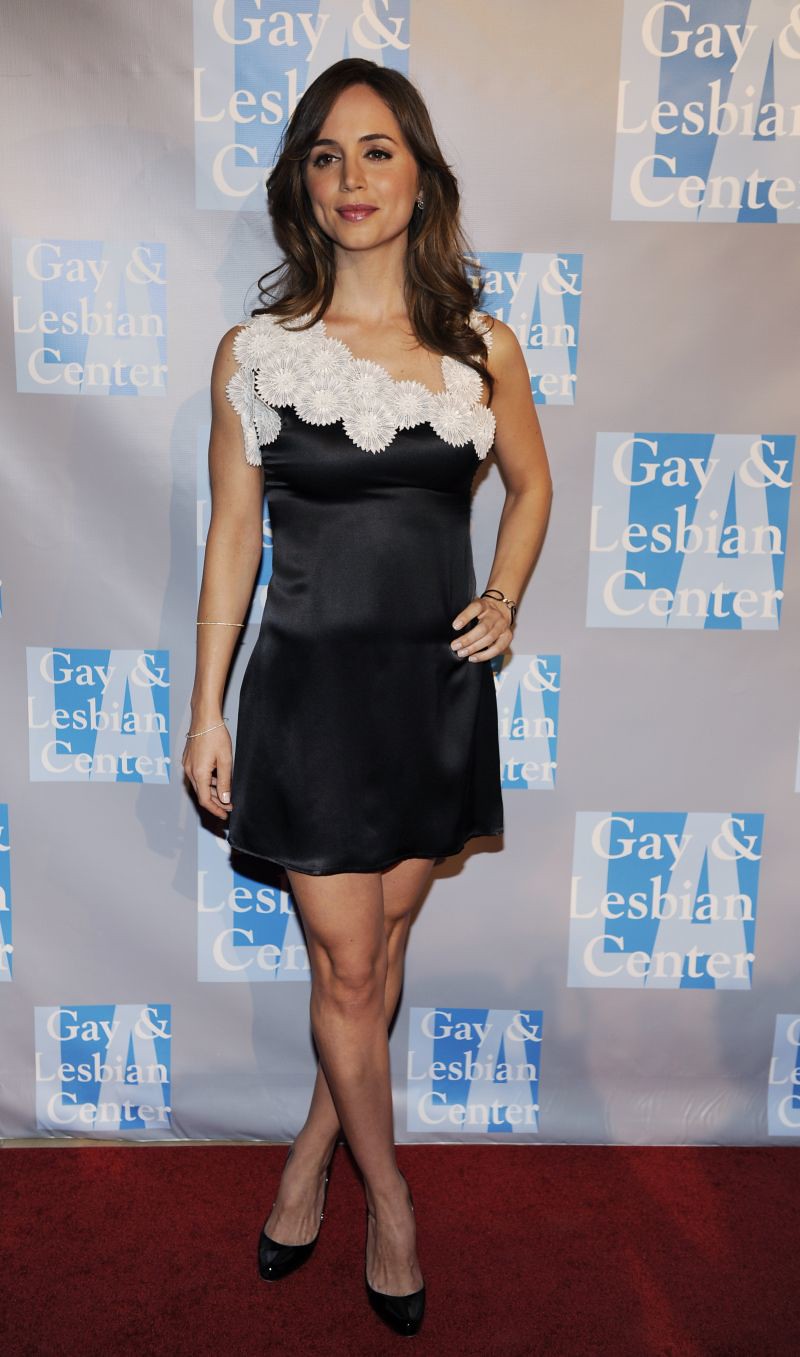A young, attractive woman, possibly in her late 20s or early 30s, poses for a picture on a red carpet. She is standing cross-legged, looking slightly off to the right of the camera with a slight smile on her face. Her shoulder-length, slightly wavy brown hair frames her face, which is adorned with a lot of makeup, including striking red lipstick. She is dressed in an elegant black dress with a white floral pattern on the top, which forms a strap that runs from her left shoulder down to her right armpit. Accentuating her outfit, she wears a silver bracelet on her left wrist and multiple gold bracelets on her right wrist. She completes her look with black high-heeled shoes. Behind her, a gray wall serves as a backdrop, featuring several rectangular signs that together read "Gay and Lesbian Center, L.A." The letters are arranged in squares with alternating gray and blue columns. The woman appears pleased to be at the event, as she confidently stands with her left hand resting on her hip.